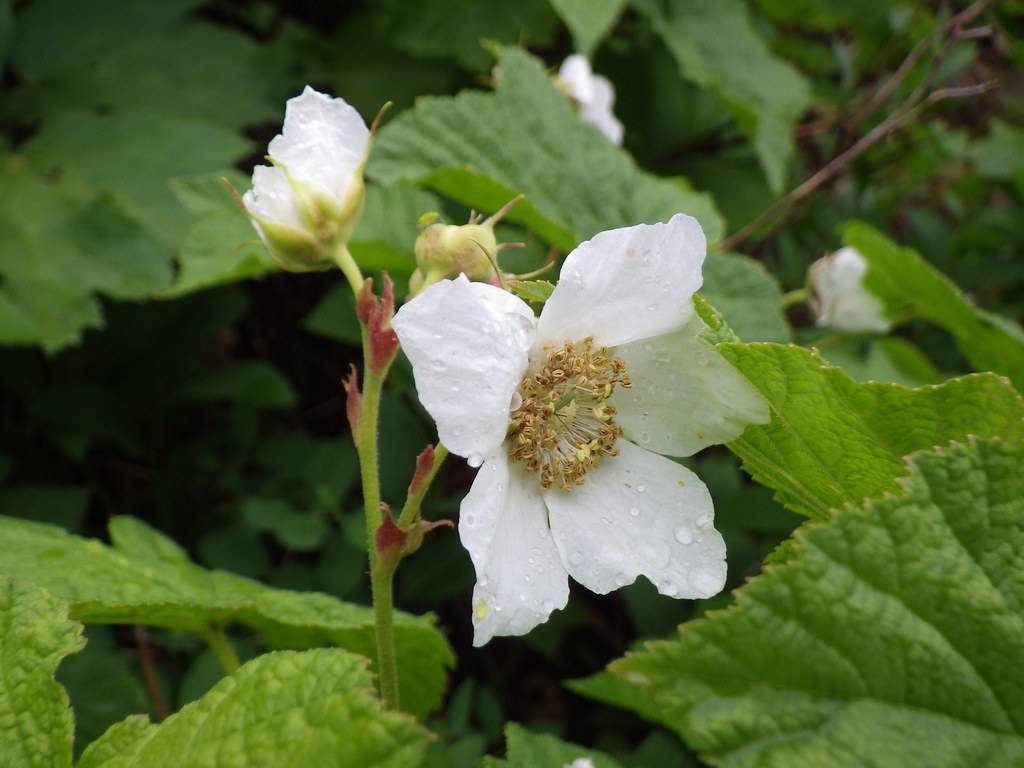A close-up, portrait-oriented photograph of a large flower with five flat, white petals, dotted with clear water droplets, possibly due to early morning dew. One petal, pointing right, is a light gray color. At the center of the flower, a cluster of yellowish-brown stamens extends outward on tiny hairs. To the left, a green stem splits, supporting a small bulb on the right and a partially hidden white flower facing backward. The background is filled with large, bright green leaves featuring rough, zigzag edges with tiny yellow points and subtle gray veins. Some stems and leaves also exhibit purple tinges and small spikes, enhancing the textured, wet ambiance of the scene.